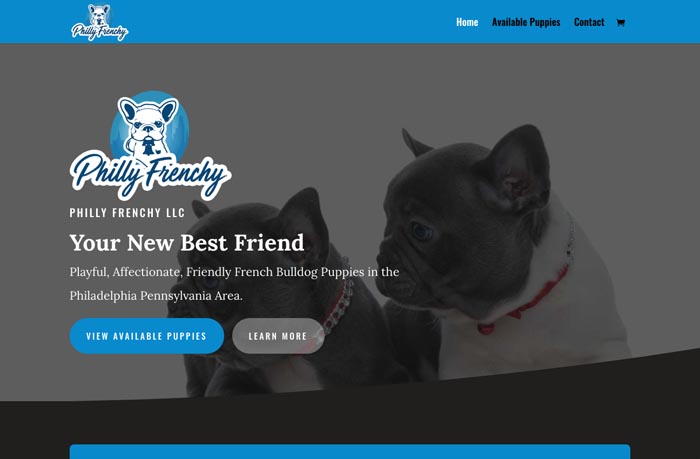The screenshot depicts the homepage of a website called "Philly Frenchie," dedicated to French Bulldogs. In the upper left corner, and prominently on the main page, sits the logo featuring the cursive text "Philly Frenchie" with capitalized 'P' and 'F'. The logo, in a blue font on a white background, is accompanied by a cartoon illustration of a French Bulldog above the text. The French Bulldog is illustrated in dark blue, matching the font color, and is set against a circular pale blue background.

Centered on the page are the words "Philly Frenchie LLC: Your new best friend," followed by a tagline describing the service: "Playful, affectionate, friendly French Bulldog puppies in the Philadelphia, Pennsylvania area." Beneath these lines, two oval buttons are displayed—one blue with the text "View Available Puppies" and the other gray with "Learn More," both in white lettering.

The website's background features a predominantly black and white photograph of two French Bulldog puppies that appear to be gray and white. The vibrant detail in the image comes from their red collars, adorned with diamond-like embellishments.